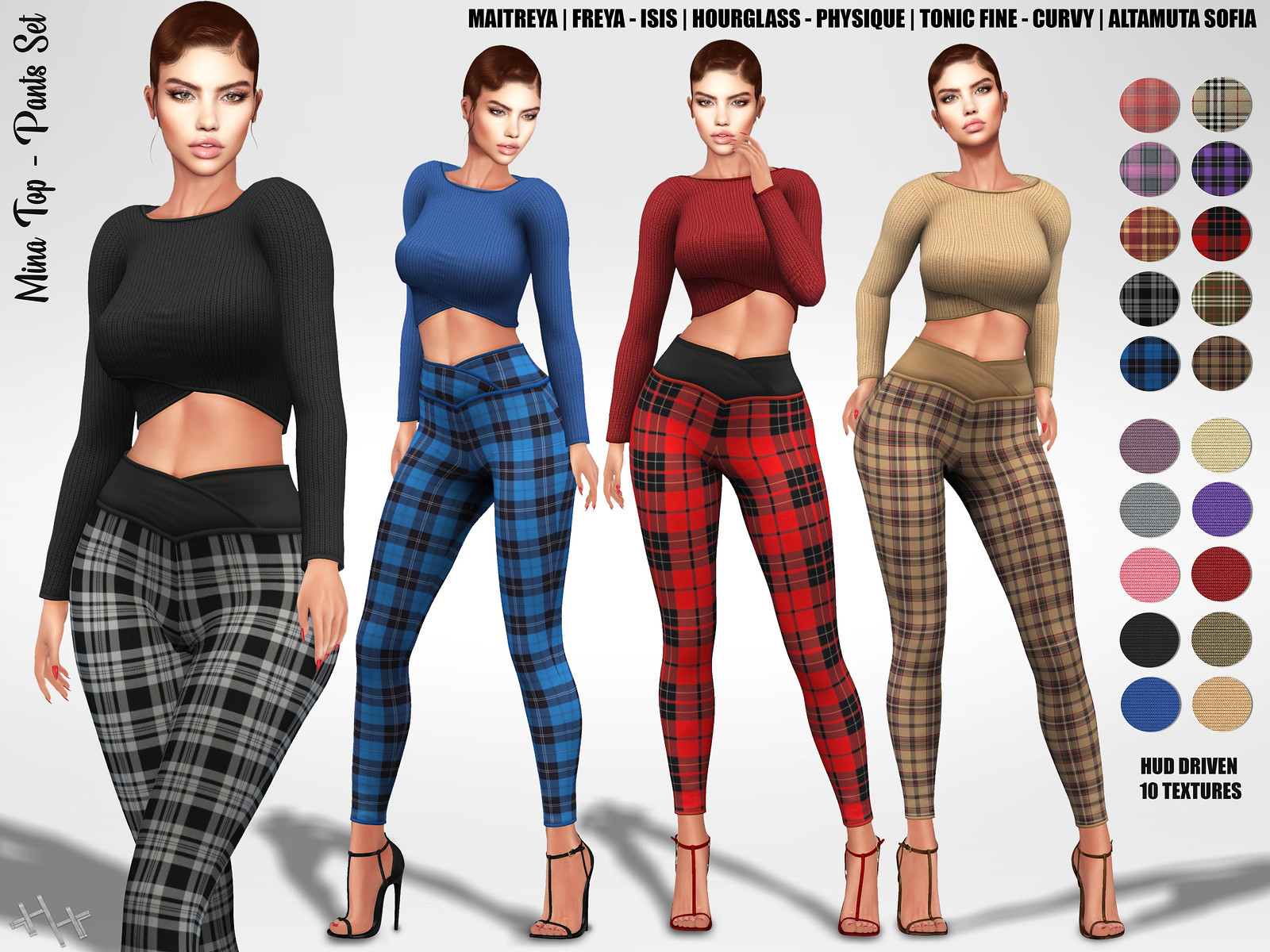The image displays four cartoonish female character avatars with identical faces and light tan Caucasian skin tones, set against a white background. They have short brown hair, makeup, and earrings. Each avatar is wearing a different colored outfit, all sporting long-sleeve crop tops and plaid pants. The first avatar on the left wears a black top with black and gray plaid pants, and only her upper body and knees are visible. The second avatar wears a blue top and blue and gray plaid pants with visible blue heels. The third avatar wears a red top and red and black plaid pants with red heels. The fourth avatar wears a tan top with tan and gray plaid pants. At the top left corner, the text reads "Mina Top, Pants Set." The top right corner lists several body types: "Maitreya, Freya Isis, Hourglass Physique, Tonic Fine Curvy, Altamura Sofia." Below this, a color palette displays various patterns and solid colors, labeled "HUD Driven 10 Textures" in the bottom right.